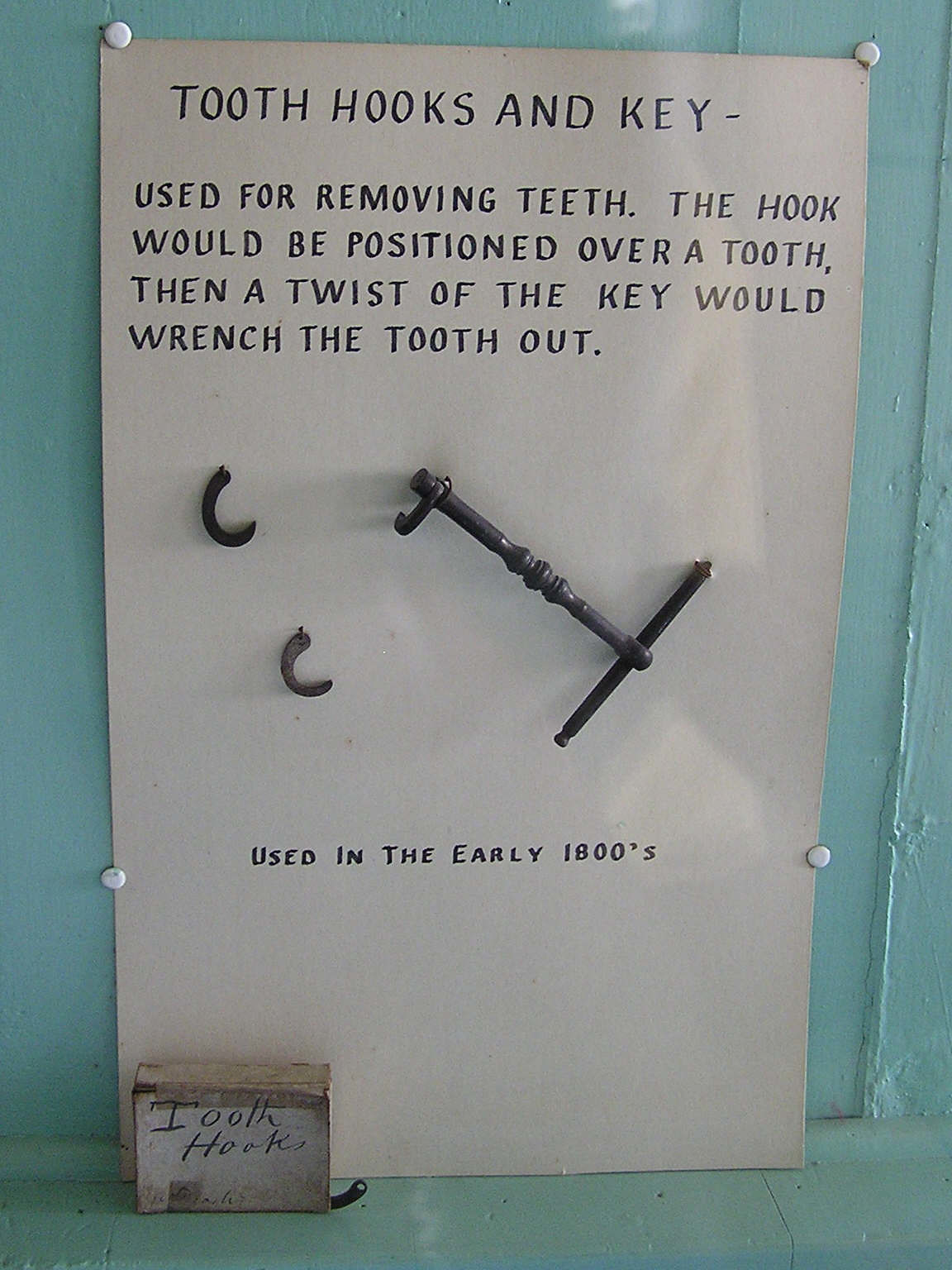The image depicts a museum exhibit featuring a historical dental instrument display. Mounted on a light blue wall, a white sheet of paper thumbtacked in four corners describes the items. The text at the top reads "Tooth Hooks and Key," followed by an explanation stating that these tools were used for removing teeth in the early 1800s. The process involved positioning a hook over a tooth and twisting a key to wrench it out. The display includes two black metal hooks, resembling the letter 'C', and a small, intricately detailed key about three inches in length. Additionally, there is a handwritten label at the bottom left of the sheet saying "Tooth Hooks." The surrounding details, such as a glossy green floor and careful mounting, suggest a thoughtfully arranged museum presentation.